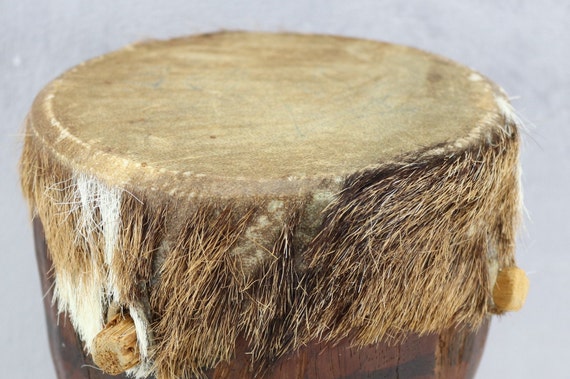This detailed photograph captures a close-up view of a hand drum set against a modeled white to gray background. The drum features a deep reddish-brown wooden body that appears well-worn and richly crafted. The top portion of the drum is covered with a smooth, beige leathery drum head, made from animal skin, which stretches halfway down the drum's body. Surrounding the drum head, patches of light brown, white, and black fur hang down, indicative of more skin left from the animal hide. Rough wooden pegs protrude slightly on either side of the drum, used to pull and secure the animal skin tightly around the drum body. White ropes run across these pegs, adding to its rustic, handmade appearance. This instrument, likely handmade and possibly of tribal origin, shows a blend of practicality and artistry, repurposing animal hides for musical expression.